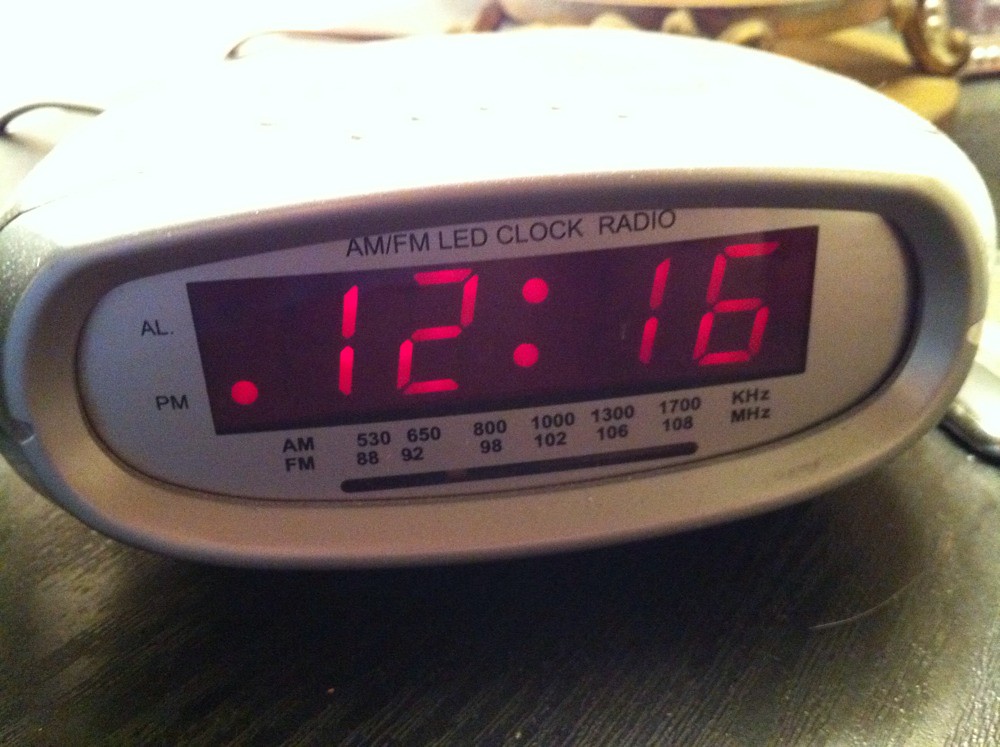A sleek digital clock radio, housed in an oval-shaped gray plastic casing with a slightly flat top, is prominently displayed. The clock body exhibits a silvery-gray color with a subtle glittery finish. Resting on a black wooden surface, which could be an end table or a desk, the clock is presently turned on. In the background, the golden base of a lamp is partially visible, adding a touch of elegance to the scene.

The clock face is flat and oval, featuring a white backdrop with a large, rectangular display that shows the digital time as "12:16," accompanied by a red colon. A small dot on the left side of the display indicates that it is PM, situated in the lower-left corner. The upper part of the clock face bears the inscription "AM-FM LED Clock Radio," positioned above the rectangular time display.

Beneath the time display, there is a section for the radio tuner. This tuner displays a range of AM frequencies: 530, 650, 800, 1000, 1300, and 1700 kilohertz. The FM band numbers are also listed: 88, 92, 98, 102, 106, and 108 megahertz. The tuning indicator is presently set between 92 and 98 on the FM band. This detailed setup demonstrates the versatility and classic design of the clock radio.